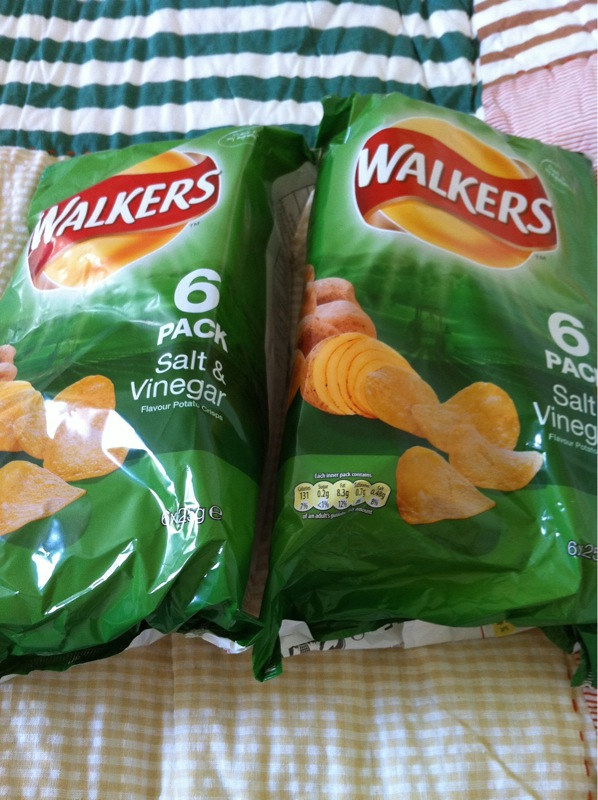The image depicts two unopened bags of Walkers' salt and vinegar potato chips. Each green bag contains a six-pack of chips. The design on the bag features images of actual chips and potatoes blending together against a multi-green background. The Walkers' logo is prominently displayed at the top of the pack, with white text on a red banner over an orange, sun-like backdrop. Nutritional information can be seen at the bottom left corner of the packaging. The bags are laying on a multicolored quilt with a variety of patterns, including green and white, pink and white, yellow gingham, and brown stripes, adding a picnic-like atmosphere to the scene. The bags appear slightly wrinkled and reflect a bit of light, indicative of the texture of the packaging material.